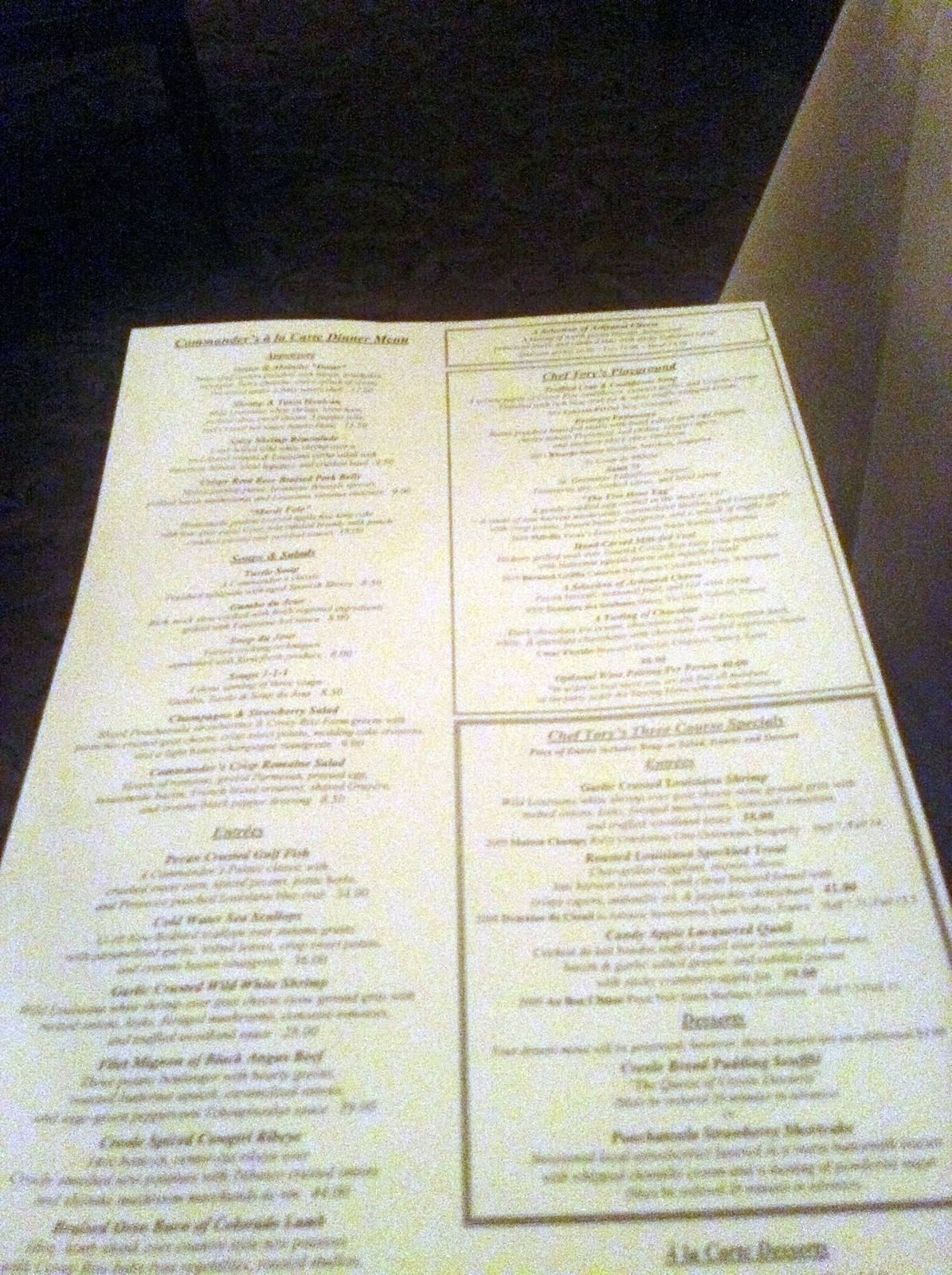The image depicts a poorly captured photograph of a restaurant menu. The photograph is blurry and of low quality, making most of the text difficult to read. The menu is notably large and tall, printed on white or ivory-colored paper. In the upper left corner, the legible text reads "a la carte dinner menu," and there's mention of "Chef Terry or Jerry's specials" and "three-course specials." The menu features sections including "Entrees" and "a la carte desserts" at the bottom. The items on the right-hand side are enclosed in text boxes. Clearly visible among the entrees is "filet mignon of black Angus beef" and something relating to "Gulf fish," though the rest remains indistinguishable. The menu appears to be propped against an arm clad in a tan or beige jacket, or possibly a chair. Due to the poor quality of the image, finer details remain elusive.